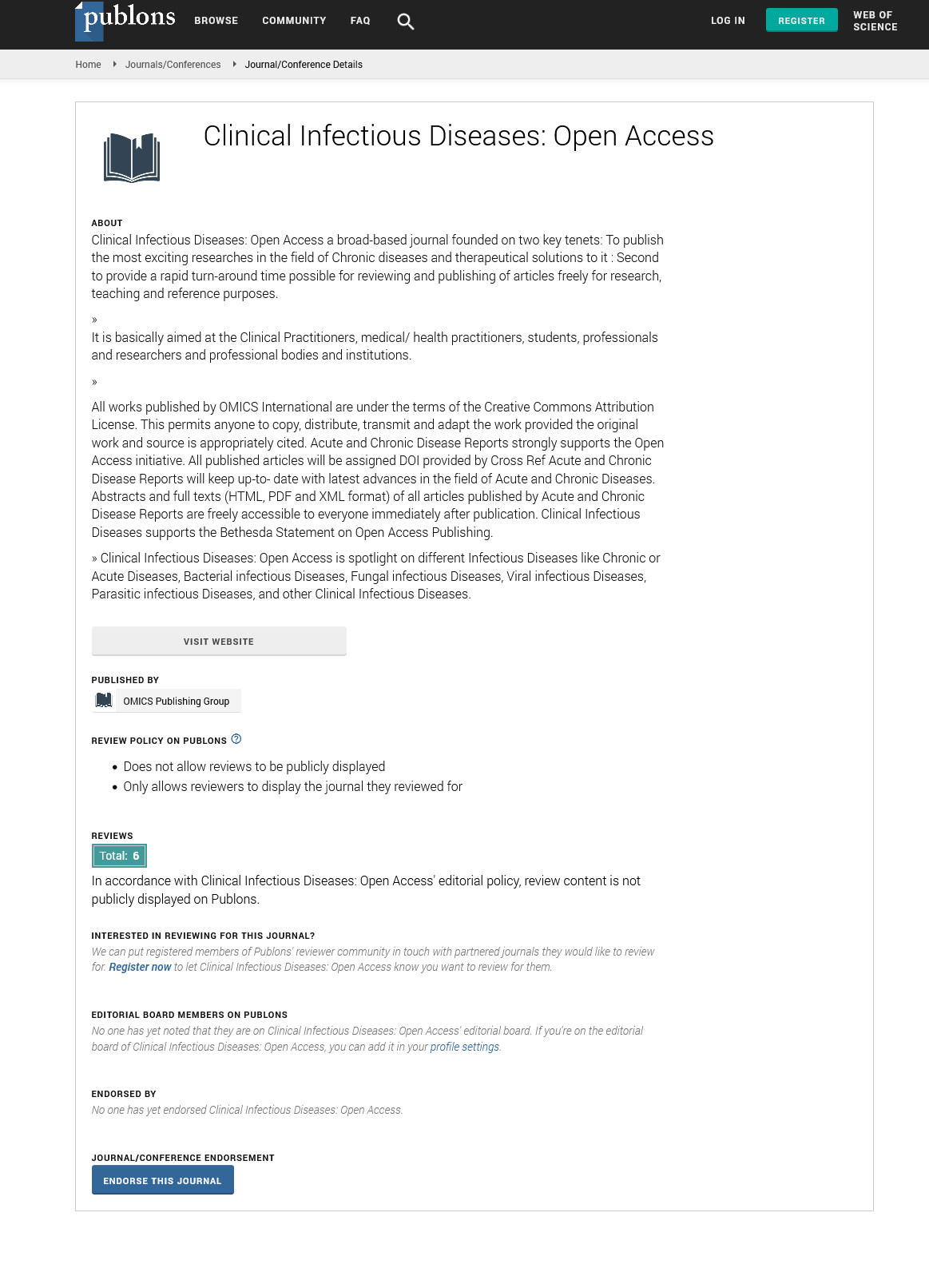**Detailed Caption:**

This image captures a webpage from Publons, a website dedicated to academic research and peer reviewing. At the top of the page, there is a navigation bar with several tabs, including "Browse," "Community," and "FAQ." A magnifying glass icon for searching is positioned next to these tabs. On the top right corner, there are options for logging in, registering (highlighted by a green "Register" button), and a link to "Web of Science."

Below the navigation bar, additional tabs are visible: "Home," "Journals / Conferences," and "Journal / Conference Details." The main content of the page is dedicated to the journal "Clinical Infectious Diseases: Open Access." The journal’s title is prominently displayed beneath an icon of an open blue book with a white bookmark.

The description of the journal highlights its focus on publishing groundbreaking research in the field of chronic diseases and therapeutical solutions. It emphasizes a commitment to rapid review and publication of articles for free access, supporting research, teaching, and reference purposes. 

Further down, the page features a "Visit Website" button, linking to the journal's publisher, Omics Publishing Group. Policy reviews for the journal can be viewed on Publons, with the page noting there are six reviews in total. At the bottom, a blue button invites readers to "Endorse This Journal."